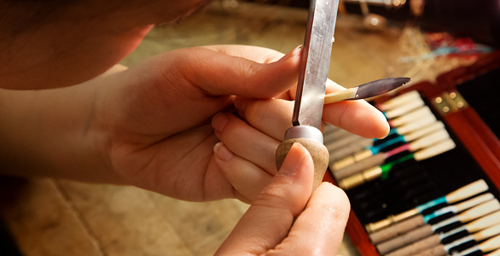The image depicts a person engaged in sharpening a cylindrical object using a metal tool with a light brown wooden handle. The right hand, which only has two fingers visible, grasps the handle of the tool, while the left hand firmly holds the object being sharpened. The bottom portion of the person’s face is visible in the top left corner, revealing short brown hair that dangles towards their chin. The setting is indoors, suggested by the artificial light. The background consists of a wooden table with a reddish-brown wooden case that has gold hinges, housing at least 20 similar tools. The scene also includes several brushes and a toolbox underneath the hands.